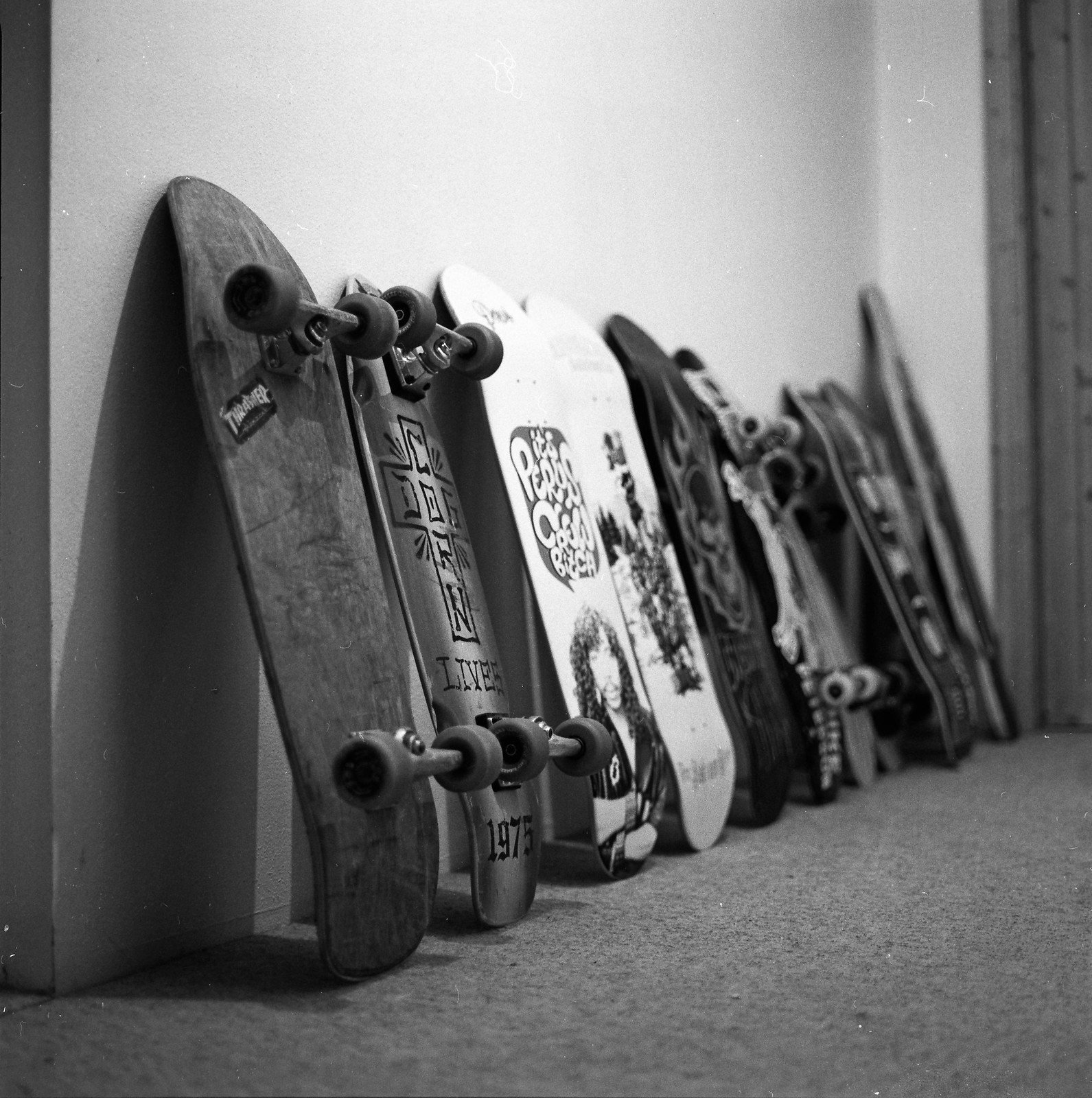This is a detailed black-and-white photograph capturing eight skateboards leaned against a grayish wall, illuminated from the center by an unseen light source, causing the wall to appear brighter in the middle. The skateboards are slightly angled toward the upper left corner of the image, which fills most of the frame. The textured, carpeted floor upon which they stand is clearly visible. To the left, the corner of the wall fades into shadow, while a wooden door frame is just visible on the right-hand side.

Most of the skateboards display their wheels, which are made of metal, with some facing the opposite direction. The boards feature a variety of decals and graffiti, although the exact details are difficult to decipher. Two skateboards in the center stand out due to their lighter color; one of these has an out-of-focus image of a person and unreadable text, while the other shows a clearer image of a person with black curly hair and some bubble letters. Another board exhibits a black-and-white skull surrounded by flames. Additionally, a skateboard on the lower bottom is marked with the design "1975" and the word "LIVES" next to a tribal cross pattern.